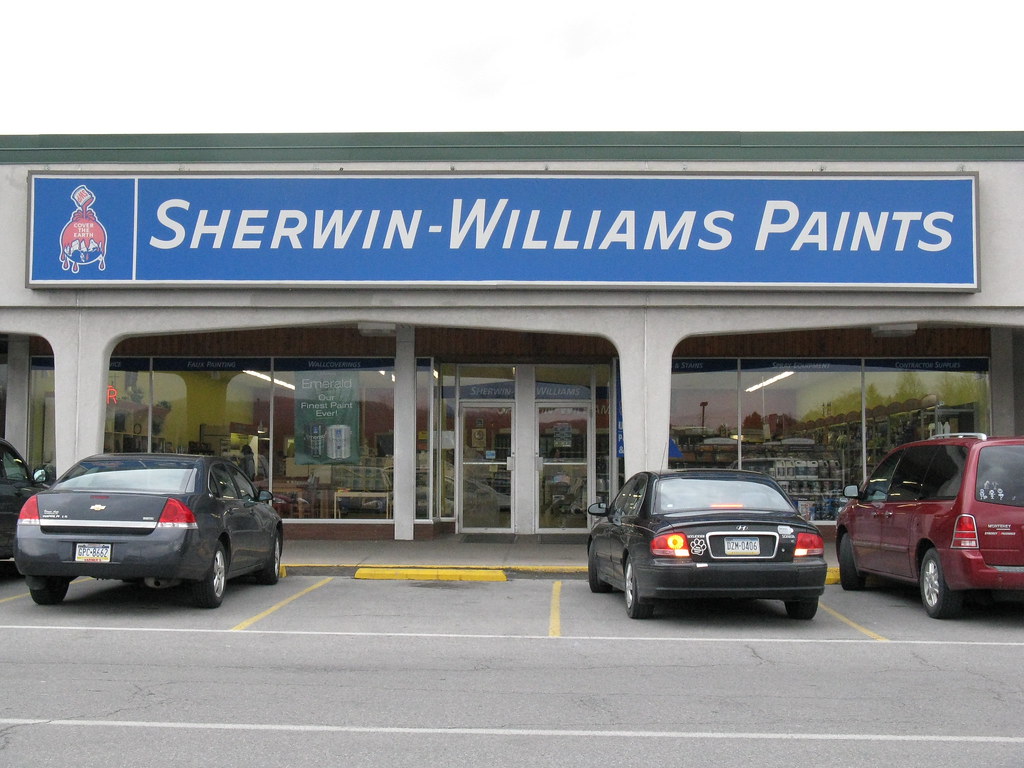The image depicts a storefront captured in a horizontal rectangular format. At the top edge of the photograph, a green horizontal line is visible, flanked by what appears to be molding. Below this line is the store's sign, a horizontally oriented rectangular sign featuring a royal blue background with capital white letters centered on it. 

To the left of the lettering is a logo, albeit somewhat hard to discern precisely. It appears to be an animated depiction of a can of red paint pouring paint over an object, with red paint drops falling from the bottom. Following a vertical white line, the sign reads "Sherwin-Williams" and "PAINTS" in white letters. The royal blue segment of the sign is bordered by a thin white edge and encased in a sleek, silver frame.

The storefront showcases its entrance with visible front doors and windows. A green sign hangs prominently in front of the windows. In the foreground, cars are parked facing the store, with their rear ends directed towards the camera. On the extreme left of the image, the edge of a dark grey car is partially visible, and next to it is a full view of a grey car. There is a vacant parking space followed by a car that resembles a sports car, partially highlighted by its illuminated taillight. Further to the right, part of a red vehicle, likely an SUV or minivan, is discernible. The concrete pavement of the parking area is apparent, with white parallel stripes running horizontally from left to right across the road.